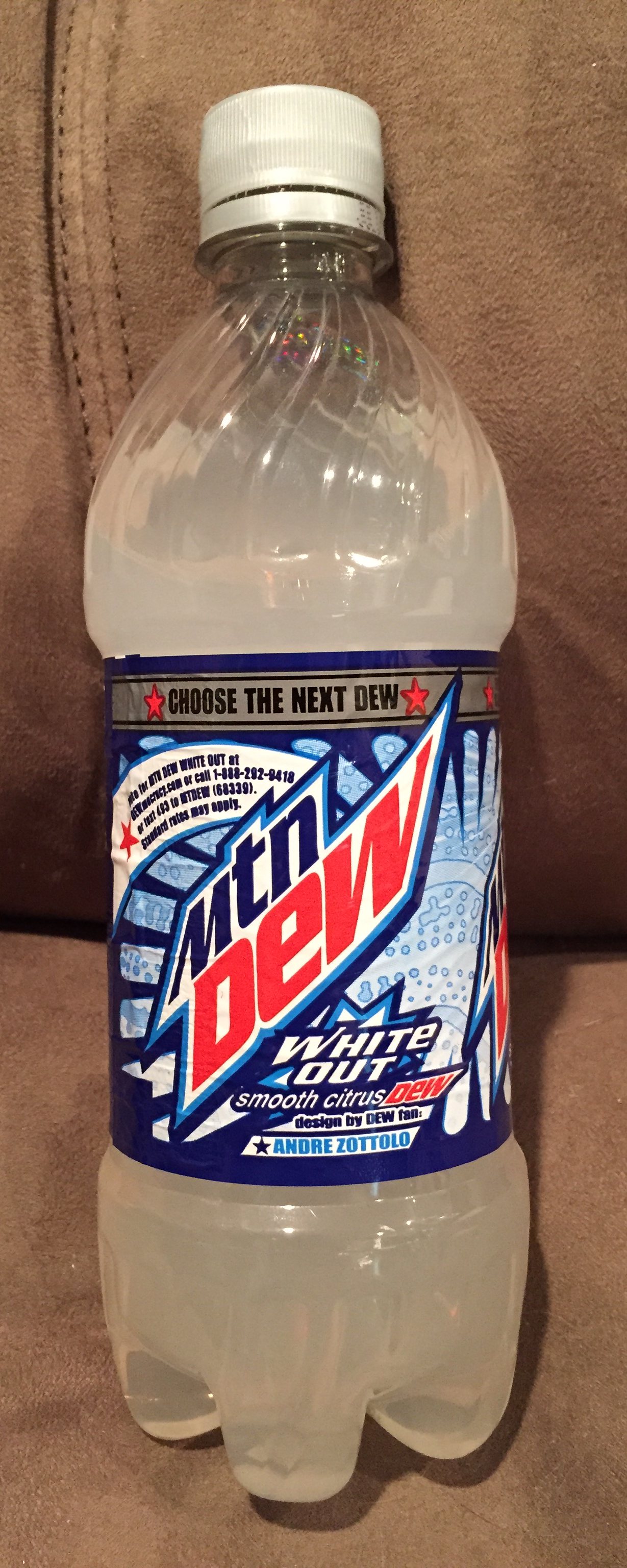The photograph features a vertically-aligned bottle of Mountain Dew White Out, resting on a plush brown couch. The bottle, which appears to be 12 ounces, is nearly full and has a white cap. The liquid inside is a clear, light grayish-white. The label prominently displays "Choose the Next Dew" with two red stars flanking the text. Below it, "MTN DEW" is written with "DEW" in red, and underneath that, the name of the flavor "White Out" is highlighted with a blue spiky star. The flavor is described as "Smooth Citrus Dew" in red text. At the bottom of the label, the designer Andre Zottolo's name is mentioned in blue text. The bottle also provides information on how to vote for the next flavor via calling, texting, or visiting the website dewmocracy.com.